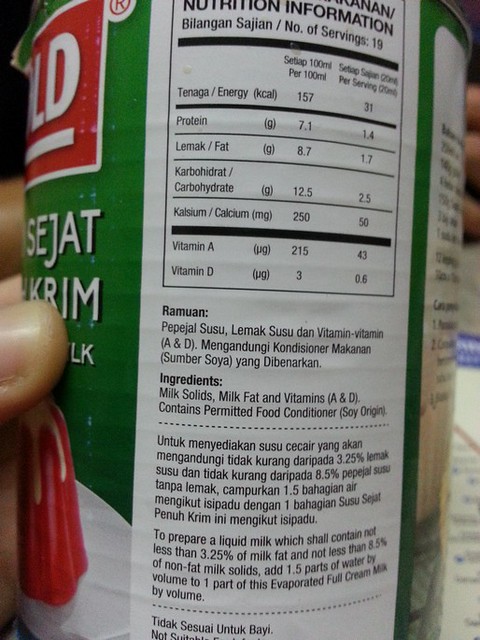The image is a close-up photograph of the nutritional information label on the side of a can-shaped food product. The text on the label is in two languages, including English. Ingredients listed include milk solids, milk fat, vitamins A and D, and a permitted food conditioner with soy origin. Preparation instructions detail how to make a liquid milk containing not less than 3.25% milk fat and not less than 8.5% nonfat milk solids, indicating this is a condensed milk product intended to be mixed to a desired consistency. The label also features an image of a red jelly with cream drizzling on top, suggesting it can be used as a topping for various foods. Additionally, the can has a green section with red lettering and symbols, and the letters "LD" and "SJAT KRIM" appear prominently. On the bottom left of the image, there's a hand holding the can, adding to the context of its usage.